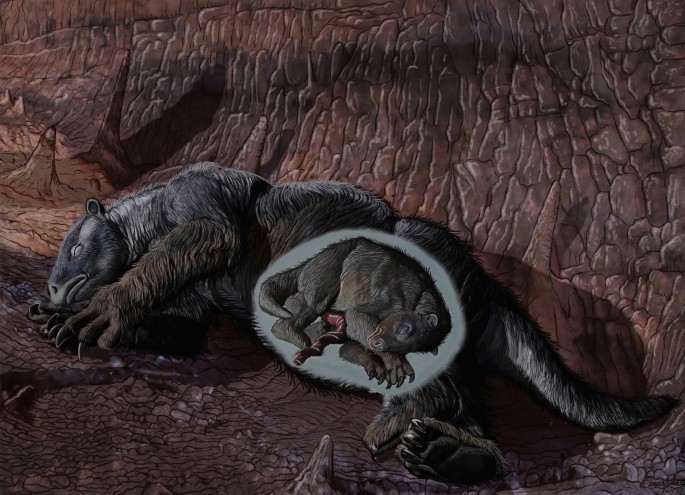The image is a computer-generated illustration of a prehistoric, sloth-like mammal sleeping inside a cave. The creature, covered in thick, coarse fur, has a gray back and brown fur on its legs and stomach. It features large bear-like paws on its back legs and claws on its front legs, and it is lying on its right side, with its thick tail stretching out to the right and its round, horse-like face with eyes closed on the left. Notably, a circular area on its stomach reveals a baby version of the animal, seemingly indicating pregnancy. The cave itself has smooth stone walls with a light brown to dark brown textured appearance, and the dark gray, pebbled floor adds to the shadowed, dim atmosphere. There appears to be a source of light in the upper left corner, possibly marking the cave's entrance, highlighting an otherwise shadowed environment. The illustration captures intricate details, from the animal’s small ear to the visible features of the unborn baby within, creating a vivid depiction of prehistoric life.